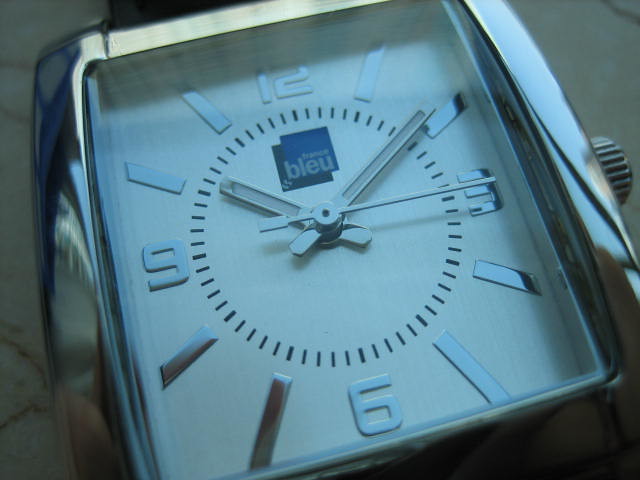The image showcases a luxurious French wristwatch named "Bleu," spelled B-L-E-U. The watch features a distinctive square face framed in elegant sterling silver. On the right side of the watch, a sterling silver tuning knob is visible, used for adjusting the dials and setting the time. The watch rests on a sleek marble surface, adding a touch of sophistication to the scene. Its dial includes three sterling silver hands: a shorter one for the hours, a longer hand for the minutes, and a thin, extended hand for the seconds. The watch face displays the numbers 12, 3, 6, and 9, while the other hour markers are denoted by simple sterling silver lines.